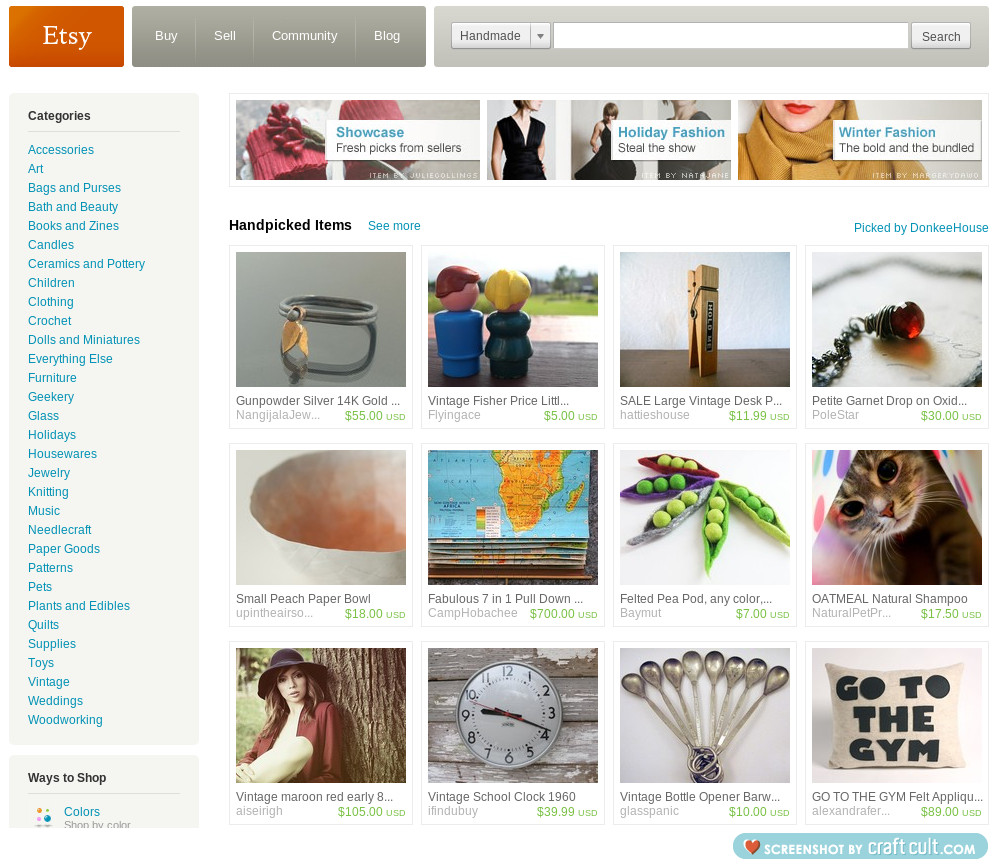This is a detailed, cropped image of an Etsy web page, focusing primarily on its layout and elements. At the top left of the page, an orange box displays "Etsy" in white print, serving as the site’s logo. To the immediate right, there is a horizontal gray navigation bar with the following categories listed: "Buy," "Sell," "Community," and "Blog." Further to the right, there is a search bar accompanied by a drop-down box on the same gray bar, set to "Handmade."

The main body of the page, featuring a clean white background, is divided into two primary sections. On the left side, a large vertical gray box labeled "Categories" at the top left lists multiple categories in blue font extending down the page.

On the right side, the page showcases various product thumbnails and categories. The page is partially scrolled down, revealing only the top halves of some images. Just below this preview, small black letters read "Handpicked items" on the top left, with a "See more" hyperlink in small blue letters to its right. To the far right, the phrase "Picked by" indicates curated selections, though the curator's name isn’t visible in this cropped image. Each thumbnail is accompanied by the price and the creator's name in gray text underneath. This detailed overview encapsulates the organized and user-friendly design of the Etsy web page.